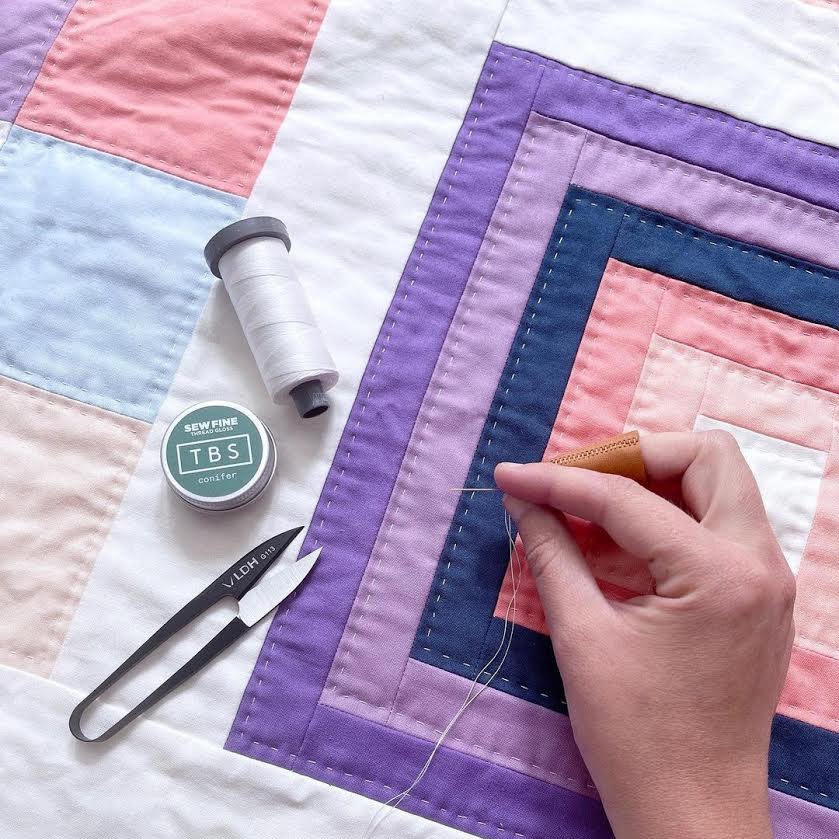This close-up photograph captures a woman with very light skin sewing patches onto a quilt, which is constructed from a series of multi-colored squares arranged in a structured pattern. The central square she is about to sew is bordered by a gradation of shades—white, light brown, pink, light red, blue, light purple, and dark purple, all set against a white background. Her middle finger is protected by what looks like a leather or synthetic thimble, and she holds a needle threaded with white thread, aimed at sewing the edges of a middle square. White thread outlines each square, emphasizing the intricate design. To the left on the quilt, we see a pair of black spring-loaded snippers and a green-labeled round canister of Sew Fine Thread Gloss, trademarked TBS and scented with conifer, alongside a large spool of white thread.